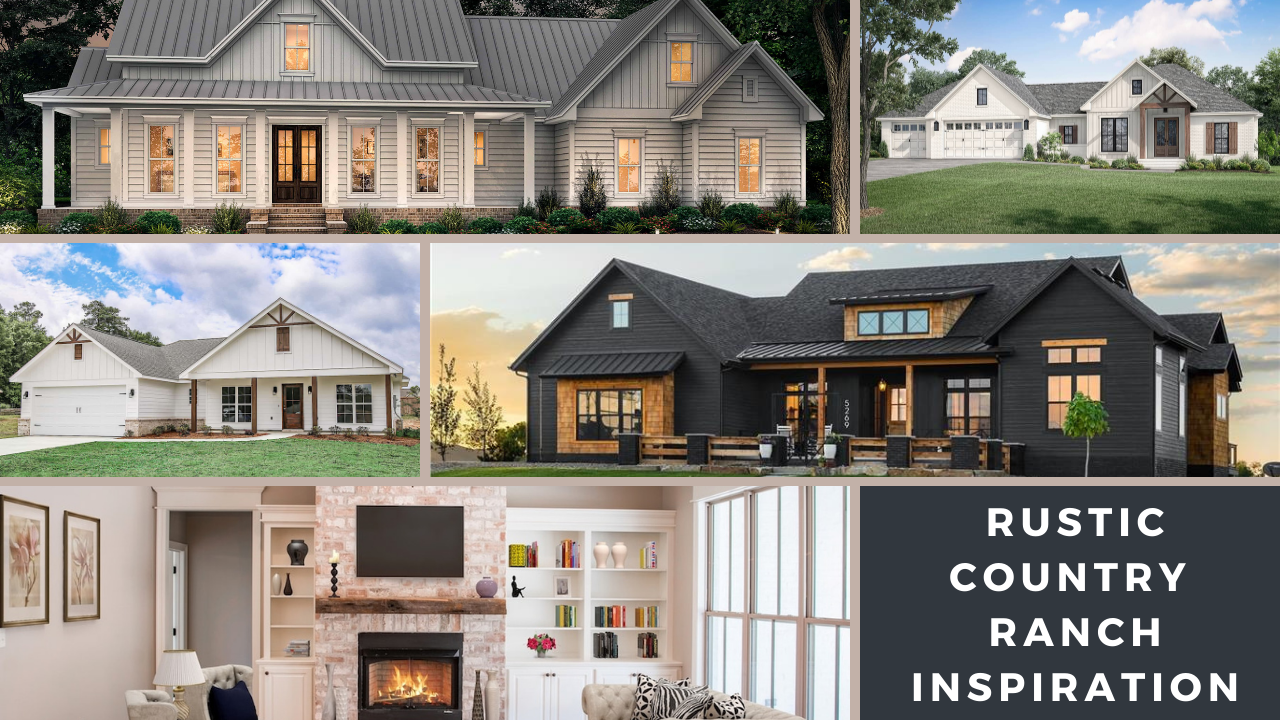The image is a horizontal rectangle collage featuring five realistic photographs of houses and a text box. The top left photograph showcases a large, two-story gray house with illuminated windows and some surrounding foliage. Next to it, on the top right, is a single-story white house with a gray roof and natural wood accents around the windows and entryway, set against a blue sky and green lawn. The middle left photograph depicts another single-story white house with similar features, including a gray roof and natural wood accents, framed by a green lawn and blue sky. To its right is a striking single-story black house with dark walls, a black roof, wooden window frames, and a patio with black pillars and light wood accents. The bottom left image reveals a cozy beige living room interior, featuring a gas fireplace, TV mounted above it, white bookcase, comfy couches, and bright windows. Over at the bottom right, a dark gray horizontal rectangle text box reads in white font: "Rustic Country Ranch Inspiration," suggesting the collage may serve as an advertisement or inspirational piece for realty or home design.